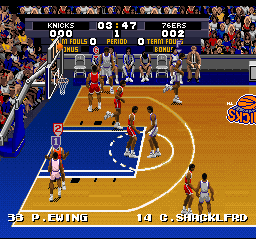Screenshot of a pixelated basketball video game featuring a matchup between the New York Knicks and the Philadelphia 76ers. The court displays players in vivid orange and white uniforms, both accented with blue trim. In the foreground, the Knicks' logo is partially visible, slightly out of frame toward the right. The bottom of the screen contains player information, notably identifying "33 P. Ewing" and "14 C. Shackleford." A scoreboard at the top indicates a score of 0-2 in favor of the 76ers, with 3:47 remaining in the first period and no fouls recorded. The bench area shows team players seated, while a colorful, generic audience surrounds the court, adding to the game's vibrant atmosphere.